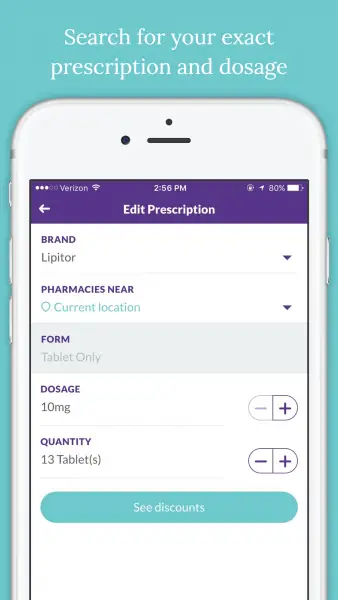The image features a light blue outline and white text at the top that reads: "Search for your exact prescription and dosage." Below the text is a white smartphone. The phone display has a status bar at the top with a purple line, showing "Verizon" on the left, the time "2:56 P.M." in the center, and a battery life indicator at 80% on the right, all in white.

Below the status bar, the screen displays the text "Edit Prescription." The next section lists "Brand" followed by "Lipitor." Under this, there is a title "Pharmacies Near" with a blue circle and the words "Current Location" in blue beside it.

Further down, there is a light-colored rectangle with the word "Form" typed within it, indicating "Tablet Only" underneath. The "Dosage" section specifies "10 mg," accompanied by a negative and positive sign to adjust the dosage. Next, the "Quantity" section lists "13 Tablets," also adjustable with a negative and positive sign.

At the bottom of the display, there is a green circle containing the words "See Discounts."